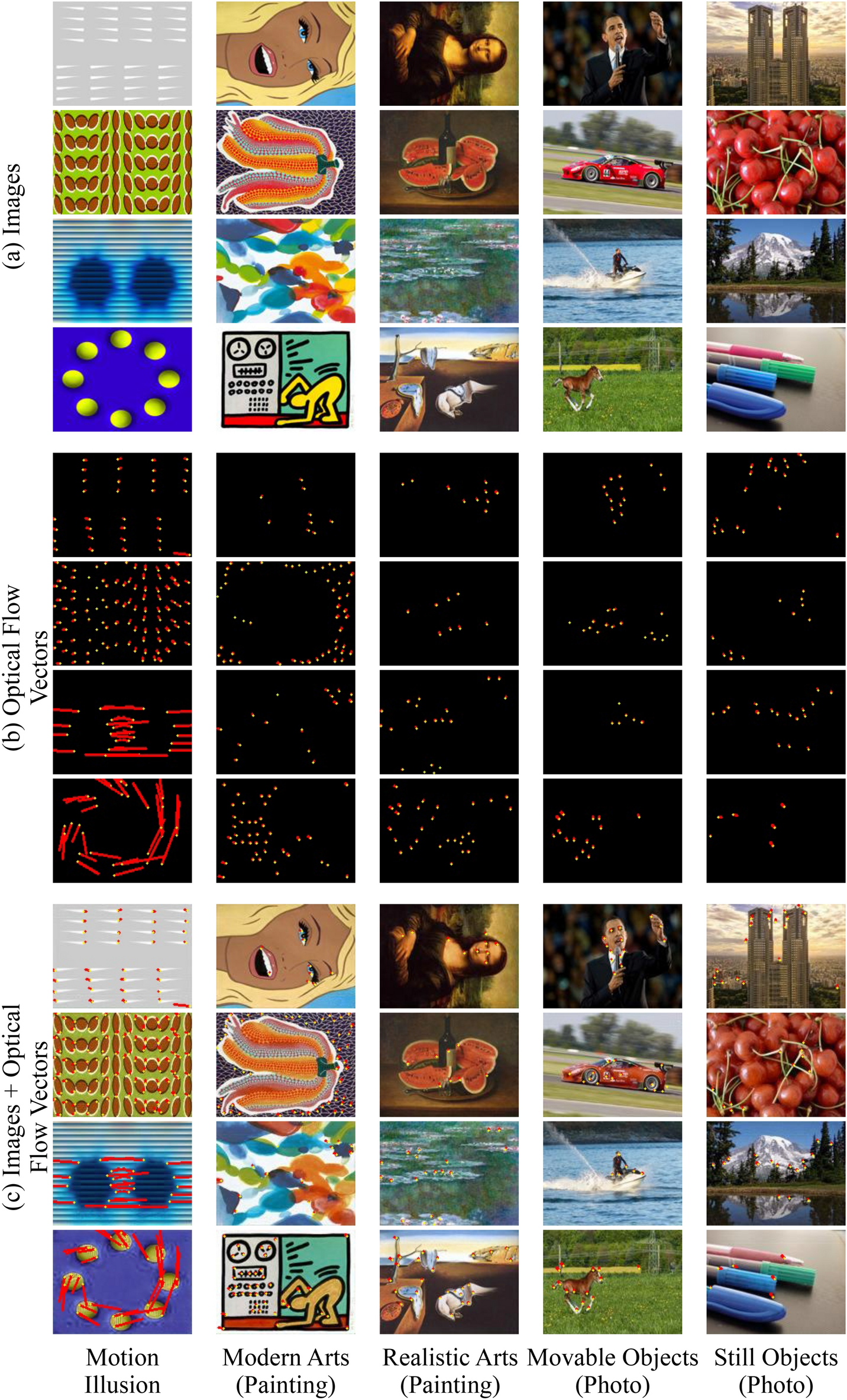The image is a detailed collage consisting of 60 small rectangular images arranged in a grid format with 5 columns and 12 rows. Each column is labeled at the bottom, from left to right, as Motion Illusion, Modern Arts (Painting), Realistic Arts (Painting), Moveable Objects (Photo), and Still Objects (Photo). The rows feature various images, including a singular gray and white square in the top left, a sideways portrait of a tan, blonde woman in the second column, the Mona Lisa in the third column, followed by a man in a suit in the fourth column, and a depiction of two towers with a tan background in the fifth column. Notably, the tenth row, fifth column has a cluster of red tomatoes. The last row's first column on the twelfth row features a purple background with circularly arranged yellow tennis balls with red lines emanating in all directions, while the fourth column in the same row showcases a young horse or foal running to the right on a grassy field. Throughout the collage, viewers can observe a mix of artistic styles, ranging from cartoony artwork to realistic photographs, capturing diverse subjects such as fruits, renowned paintings, and scenes of motion. Additional text on the image describes 'images and optical flow vectors', indicating a blend of visual themes and optical studies within the collage.